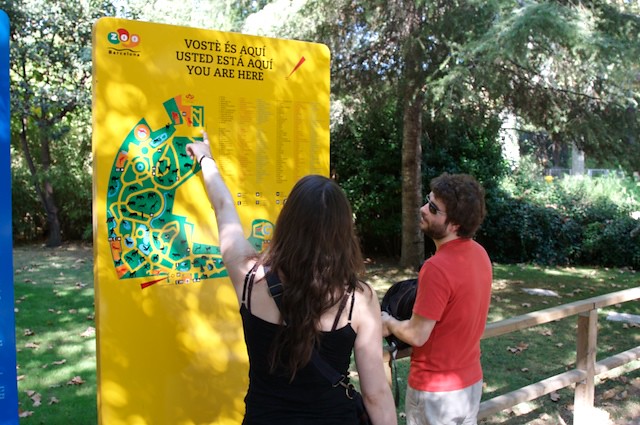The photograph features a young couple examining a large yellow zoo map signboard. The signboard has three lines of large black text in Spanish at the top, including "Usted está aquí," which translates to "You are here," alongside a similar phrase in another language. On the left side of the signboard is the actual map, depicting outlines of various creatures, while multiple lines of text are visible on the right side. The setting suggests it's a lush, greenery-filled environment, possibly the Barcelona Zoo, as indicated by the signboard.

The woman, seen from waist up, is wearing a thin, black strapped, sleeveless top with visible underlying clothing straps. Her left arm, adorned with a wristband, is raised as she points to a specific area on the map. Beside her, the man, also visible only from the waist upwards, is dressed in gray pants and a short-sleeved red shirt. He has short hair, sunglasses, a short trimmed beard, and holds a backpack which is resting on a wooden rail fence. The fence is composed of wooden planks, adding to the rustic and natural feel. The couple appears to be deeply engaged with the map, planning their next move in the expansive zoo grounds.